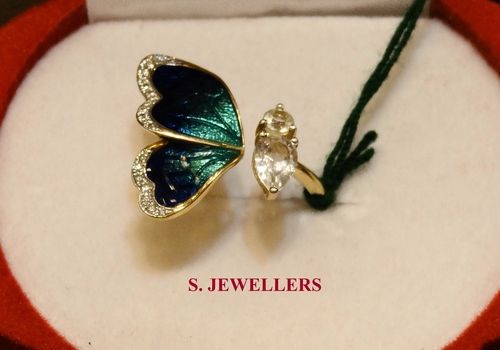The image captures a close-up photograph of intricate jewelry housed in a small jewelry box. The box features a white or light tan felt material center and has foamy red accents on its sides and corners. At the bottom of the image, in red text, it reads "S. Jewelers."

Centered in the box is a gold ring, which is not a complete circle and is adorned with a series of jewels. It has an oval-shaped diamond as its main centerpiece, with a circular diamond positioned on top of the oval. Extending to the left of the ring is a separate yet complementary piece of jewelry in the shape of butterfly wings. This secondary piece has an ombre effect with its green color and is detailed with gold outlines around each wing. Tiny diamonds border the edges of these wings, with the upper wing being slightly larger than the lower one. The precise connection between the two pieces of jewelry is ambiguous, heightened by a black yarn tied to the gold ring, trailing down from the upper right corner of the photo to the jewelry itself.

Together, these pieces showcase a delicate blend of elegance and complexity, with sparkling diamonds, rich green hues, and finely crafted gold settings, all elegantly presented by "S. Jewelers."